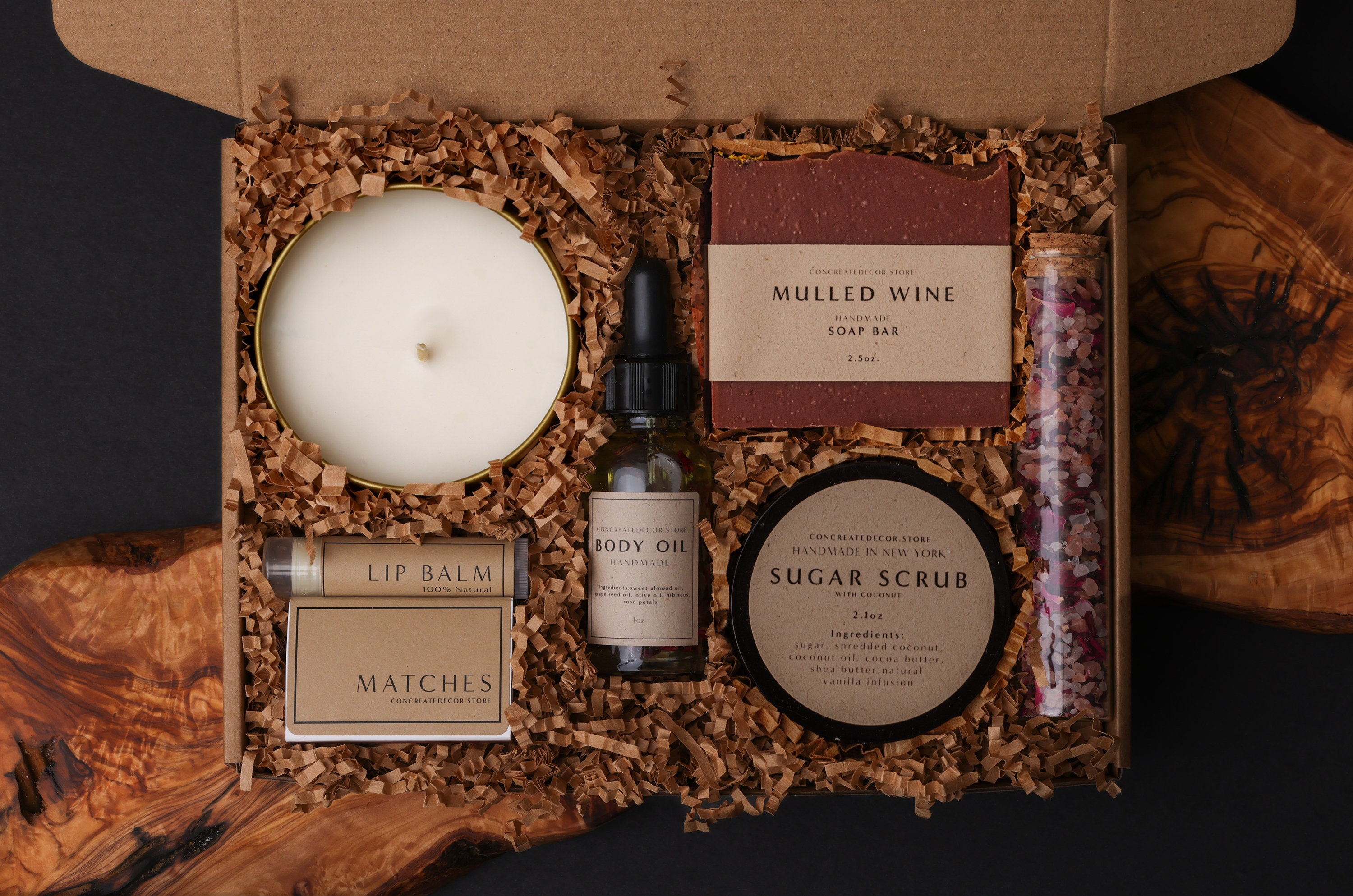This is an overhead color photograph of an elegantly presented gift box, likely from a specialty store. The box is made of corrugated brown cardboard with its lid lifted, revealing the underside of the lid at the top of the image. Inside, various body care and home goods are nestled in shredded, zigzag-style brown paper. 

In the upper left corner, a white candle in a gold cup is visible, with its wick centered. The upper right corner holds a soap bar labeled as "Mulled Wine Soap Bar." The lower left section features a tube labeled "Lip Balm," with a box of matches below, presumably for the candle. Centered in the box is a bottle with a black eyedropper top, labeled "Body Oil" with some smaller, unreadable text. A package labeled "Sugar Scrub" is situated in the lower right corner. 

Additionally, on the right side, there is a glass tube—or test tube—filled with multicolored crystals and capped with a cork. The background is a black table with a wooden resin accent, enhancing the presentation of this luxurious gift box.